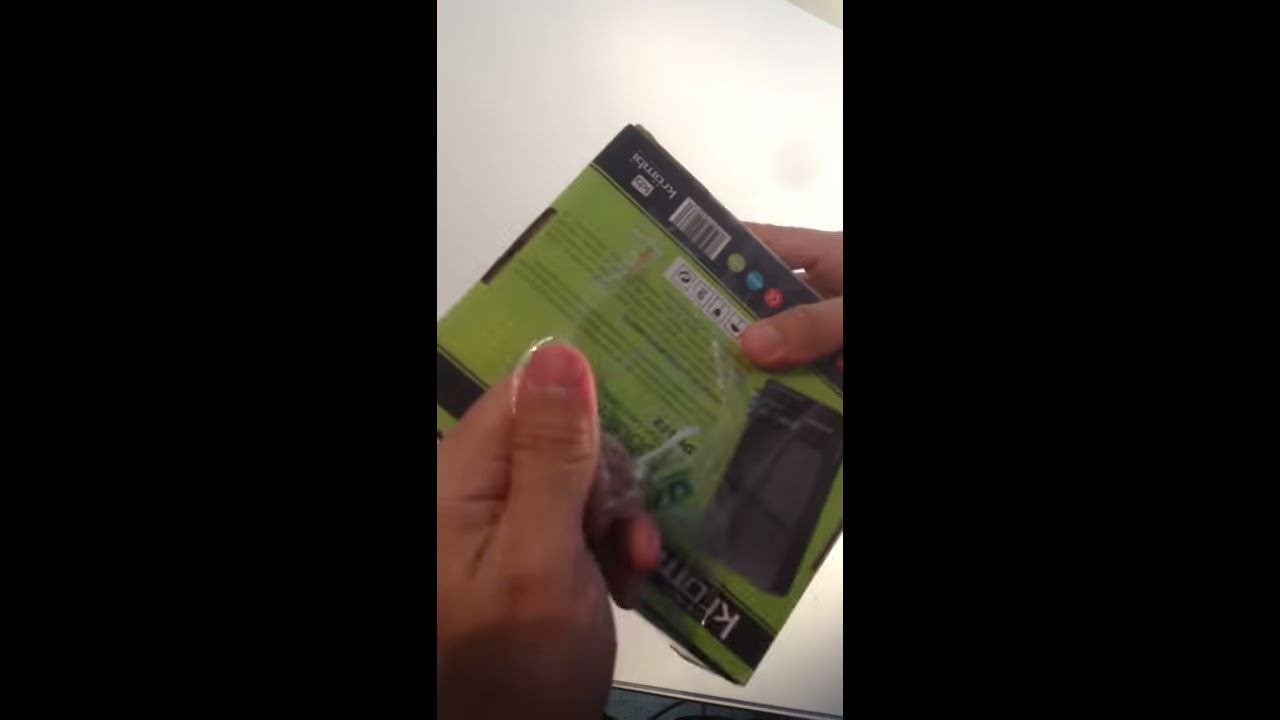In the image, two hands are interacting with a small, light green rectangular package that has black borders. The background of the picture is white, while the left and right thirds of the image are filled with black bars. The left hand, which is brownish with short nails, is primarily visible through the thumb pressing against the object, while the rest of the hand is more relaxed. The right hand firmly grips the package. The package is depicted upside down with a barcode located at what appears to be the top of the photo and a series of three dots colored green, blue, and red nearby. Some lines of upside-down text are visible, though not legible. A picture on the box suggests it might contain a phone or a charger with associated cords, hinting at an electrical apparatus.